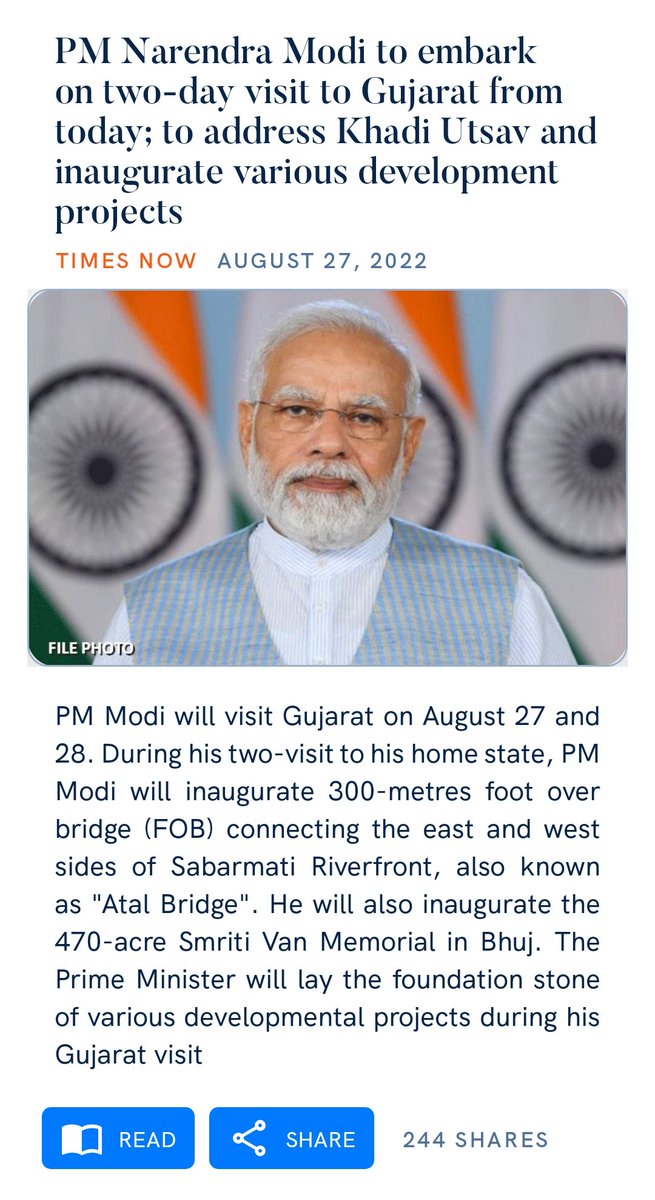**Caption**

Prime Minister Narendra Modi is set to embark on a two-day visit to Gujarat starting August 27th, 2022. He will address the Gandhi Utsav and inaugurate several development projects. The event is being covered by Times Now. In a file photo, PM Modi is pictured with gray hair, a gray beard and mustache, gray eyebrows, and glasses. During his visit, PM Modi will inaugurate a 300-meter foot overbridge, known as Atal Bridge, connecting the east and west sides of the Sabarmati Riverfront. He will also inaugurate the 470-acre Smriti Van Memorial in Bhuj. Additionally, the Prime Minister will lay the foundation stone for various developmental projects. (File Photo, August 27th, 2022, Times Now, 244 views)